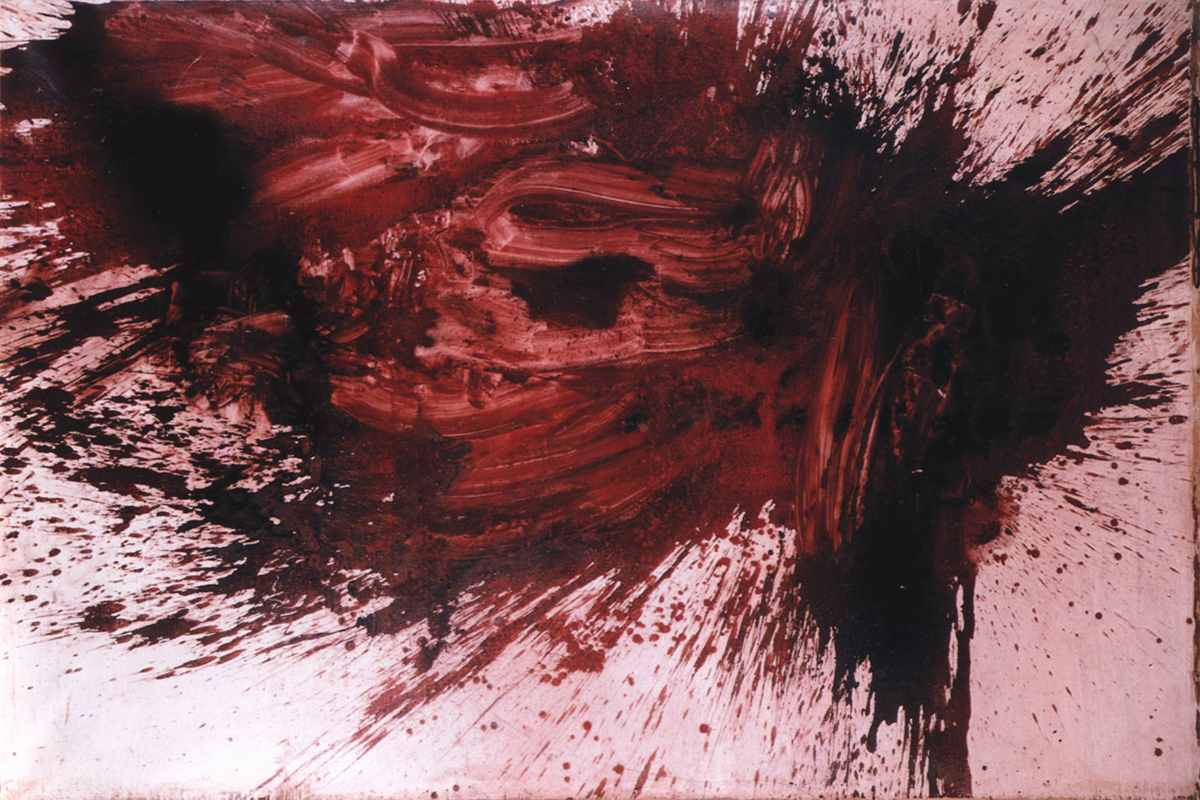The image showcases an abstract painting on a white or slightly pink-tinged canvas, featuring chaotic and aggressive brush strokes and splatters. Predominantly, the painting consists of dark red and deep, fresh blood-like colors, with parts that extend to a reddish-brown or almost black hue, particularly towards the edges. The central section of the artwork reveals intense brushwork, transitioning from deep red to darker tones that almost seem congealed or dry, giving a textured appearance. The paint appears to have been thrown on, creating explosive and disordered splashes and dots, especially around the periphery, adding to the dynamic and visceral quality of the piece.